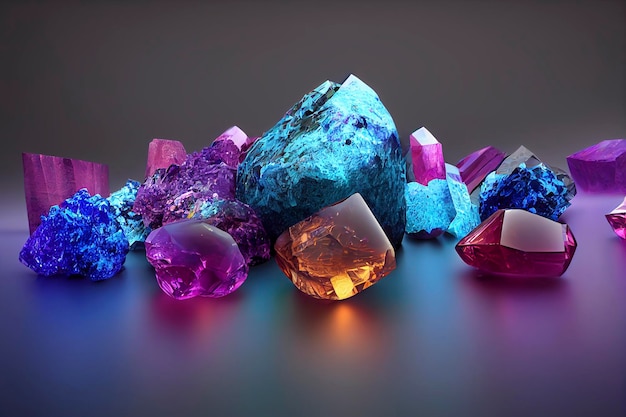The photograph showcases a meticulously arranged collection of various gemstones and rocks on a shiny, horizontal surface. Central to the composition is a distinct orange gemstone, rounded at the base and tapering to a point at the top. To its immediate left is a similarly cut purple gemstone, and to its right lies a jagged-edged red stone, potentially a ruby, with its jagged side facing left. Flanking the central stones are two blue rocks: one situated behind them and another to the left of the purple gemstone.

In the backdrop, a large, neon aqua-colored rock stands out prominently amidst a series of less defined rocks shrouded in a light fog. This ensemble is set against a neutral gray background, suggesting the possibility of a digital 3D render. The array of colors within the gemstones includes hues of blue, turquoise, yellow, and purple, all displayed in a horizontal alignment across the image. This careful positioning enhances the visual appeal of the photograph, highlighting the unique characteristics and vibrant colors of each gemstone and rock.